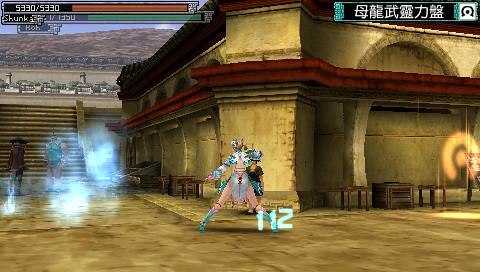This is a detailed screenshot from a video game, capturing a dynamic moment during a battle. At the center, a formidable woman resembling a Xena-like warrior stands poised, her outfit an intricate blend of blue knee-length boots, pinkish legs, a white top, and a grey midsection. She also features sleeves adorned with blue and white armor. Behind her, a figure in black is partially visible, seemingly cowering for protection. The woman stands on a golden-brown flooring in front of a tan-stone building adorned with gold and light brown columns and a distinctive red cement-like structure halfway up, topped with a black roof. 

In the background to the right, there is a yellow target-like light projected onto the building. To the left, a bluish cloud-like figure and three white and blue ghostly projections are visible. Among these, two warrior-like creatures can be seen: one dressed entirely in brown with a hat and double faces, and another reminiscent of Mr. T, sporting blue shorts and a top, with bulging arms and legs. A grey stairwell ascends behind these characters, leading to a distant cityscape with muted shades of light tan and brown buildings and mountains.

Just above the image, a health bar depicted in orange and a green XP bar are evident, displaying the accumulative scores in light blue and the number “5330/5330”. Alongside this visual, it says "SHUNK" below an Asian character. Off to the right of the warrior woman, a prominent yellow circle with a dot inside is visible, possibly indicating a target or focal point in the game. Additionally, the number "112" in light blue is written next to her right foot. The top right corner of the image features some Asian characters, underscoring the game's narrative or combat elements.